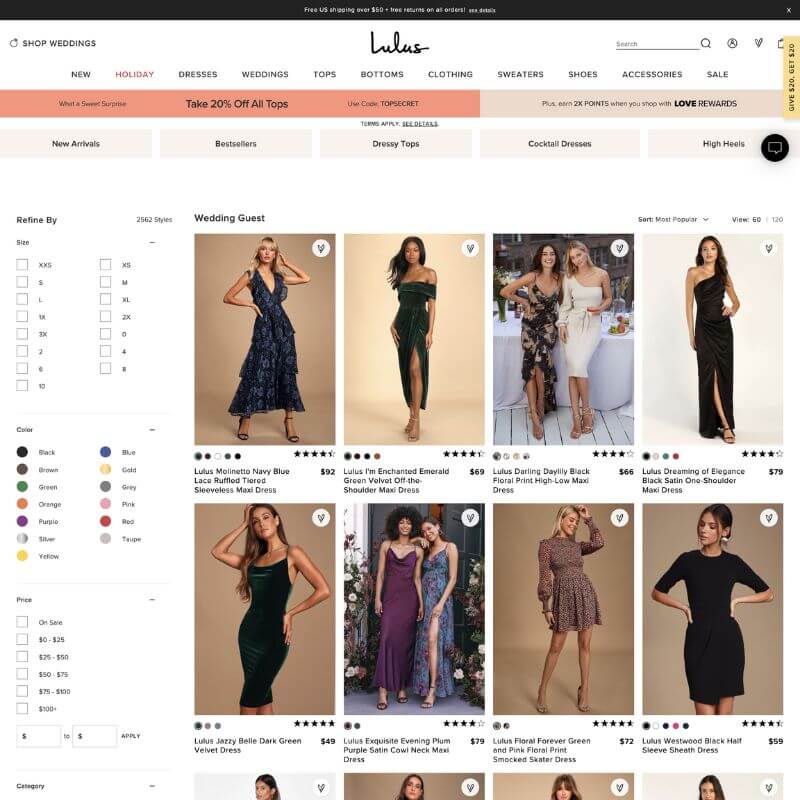The image is a detailed snapshot of Lulu's clothing website. At the top of the webpage, there's a black rectangular banner featuring white text that reads, "Free U.S. Shipping Over $50, Free Returns on All Orders. See Details." Below this banner, the website's navigation area showcases clickable rectangles in varying shades of peach and tan.

On the left side of the page, there is a section titled "Shop Wedding," indicating the collection's focus. This section displays eight images of women dressed in elegant attire. Although these dresses are not wedding gowns, they are suitable for bridesmaids or formal events.

To the right of the main content, there's a refining tool allowing users to filter their search results by size (ranging from XXS to XL), color, and price. The core of the page highlights stunning models wearing beautiful, sophisticated dresses, encapsulating the brand's stylish offerings.